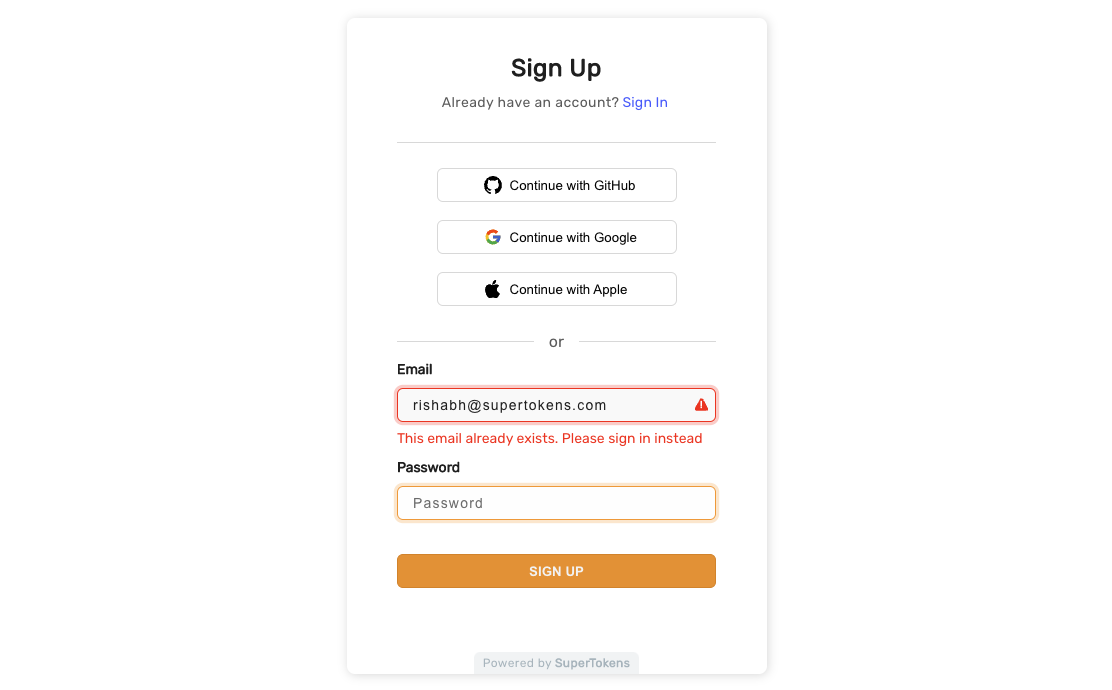A screenshot from a cell phone displays a sign-up page with a stark white background and black text that reads "Sign Up." Below this, a smaller line of text asks, "Already have an account?" followed by a blue link saying "Sign In." A faint gray line separates this section from three horizontally-aligned rectangles featuring icons on the left: a cat silhouette for "Continue with GitHub," the Google "G" for "Continue with Google," and a black apple with a bite out of it for "Continue with Apple."

Another faint gray line separates the next section, where the word "or" appears centered above a new input area labeled "Email." An email address, "rishabh@supertokens.com," has been entered into this field. Below the email, red text warns, "This email already exists, please sign in instead." This entire error message and input area is outlined with a red rectangle, featuring a red triangle with a white exclamation point next to the message.

Further down, the word "Password" appears above an orange input box where users can type their password. Finally, an orange "Sign Up" button is prominently displayed at the bottom.